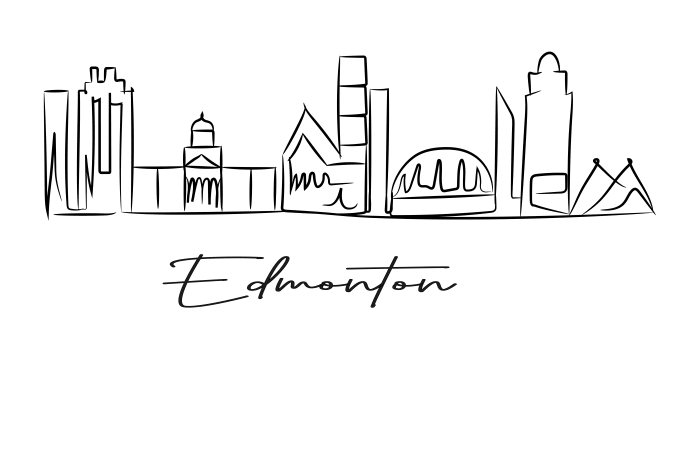This black-and-white line drawing depicts a simplistic and varied cityscape of Edmonton, Canada. Rendered in a minimalistic style with black pen on a white background, the drawing features an assortment of five distinct buildings arranged in a straight line from the left to the right. These structures include a taller building with two chimneys, a tent-like structure, a pointed building resembling either a Capitol building or a church, a dome-shaped building akin to a civic center or coliseum, and finally, a large building with two triangular forms at the base. Beneath these buildings, the word "Edmonton" is inscribed in penmanship at the bottom center of the image, suggesting these are representative landmarks of the city. The entire piece embodies a simple yet effective portrayal of the skyline, emphasizing clarity and a direct visual impression.